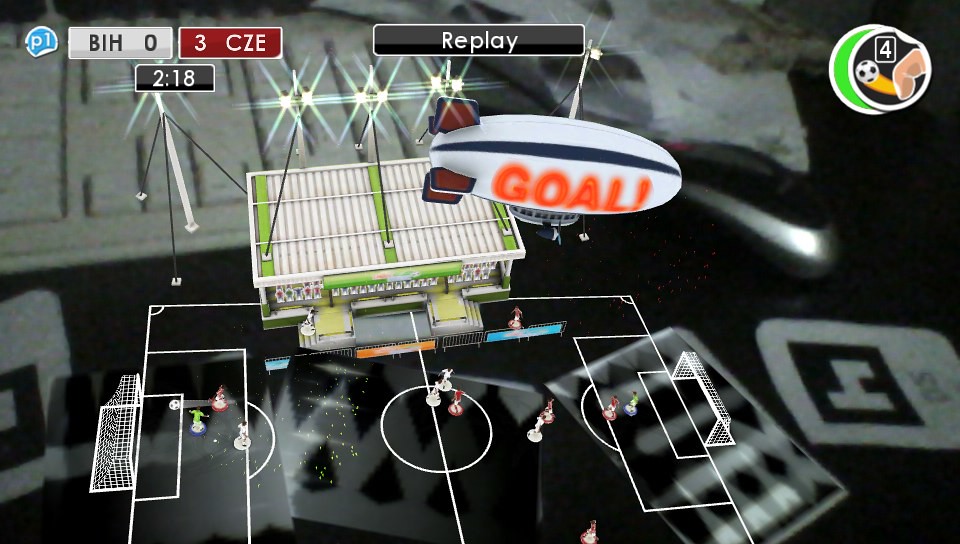The image portrays an aerial view of a video game-like soccer field, presenting a distinct, stylized appearance. At the top center of the scene, slightly to the side of the field, stands a small stadium entranceway, welcoming spectators to the virtual arena. The field is meticulously laid out with easily identifiable goalposts situated on both the left and right ends. Dominating the center of the pitch is a conspicuous white circle, marking the spot for kick-offs.

A striking feature in the image is a hot air balloon, floating above the field and displaying the word "GOAL" in vibrant, fluorescent orange glowy letters, adding an element of dynamic excitement to the scene. Additionally, in the upper left corner, tall stadium lights are visible, poised to illuminate the field during nighttime matches. The overall aesthetic captures the essence of a lively and immersive sporting event within a digital domain.